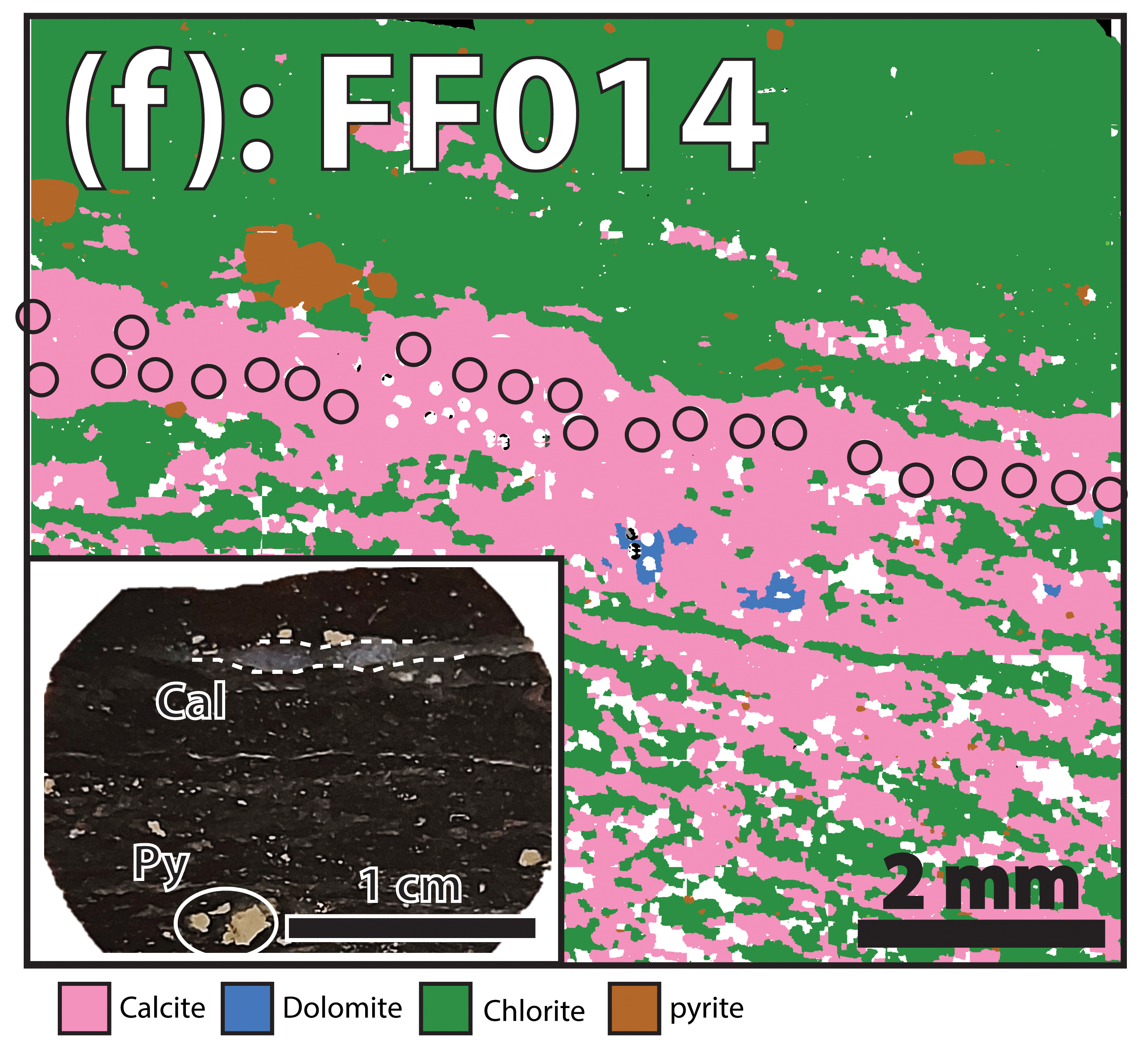This is a detailed color-coded computer-generated map, likely depicting geological formations. At the top of the image, green blotches form a distinct layer interspersed with small orange and pink specks, identified as chlorite. Directly below, a prominent layer of solid pink with patterned circles stretches horizontally across the image, representing calcite. Scattered within this pink layer are smaller green, white, and blue elements, with the blue indicating dolomite. In the bottom left corner, a white square features a black circle labeled "CAL" and "PY," the latter representing pyrite. On the bottom right, a scale indicates measurements, with 2mm showing the distance between elements in the image. The entire visual is annotated with labels including “(F:FF014),” providing additional identification markers.